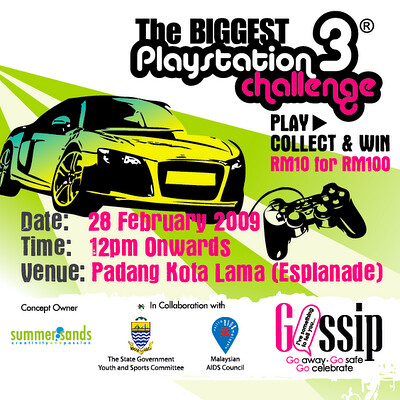This is a detailed advertisement for the biggest PlayStation 3 challenge, set against a white background with vibrant green rays or stripes extending from the left to the right. The dominant colors include black, white, pink, and golden, with hints of blue and green contributing to the vivid aesthetic. At the top, bold black text announces "The Biggest PlayStation 3 Challenge," with the word "challenge" standing out in red. Below this headline, a stylish sports car, resembling an Audi GT, appears in clip art form with a black outline and complementary hues, including green and yellow shading.

Accompanying the car graphic is an iconic black PlayStation controller clip art. The advertisement details key information: the date, February 28, 2009; the time, starting at 12 p.m. onwards; and the venue, Padang Kota Lama Esplanade, in purple text. The tagline "Play, Collect, and Win" is prominently displayed along with the offer "RM10 for RM100."

At the bottom right, in green and blue text, the message reads, "Gossip, Go Away, Go Safe, Go Celebrate," encapsulated within a text box. Concept ownership is attributed to Summer Sands, and the collaboration partners are listed as the state government youth and sports committee and the Malaysian AIDS Council, each accompanied by their logos.